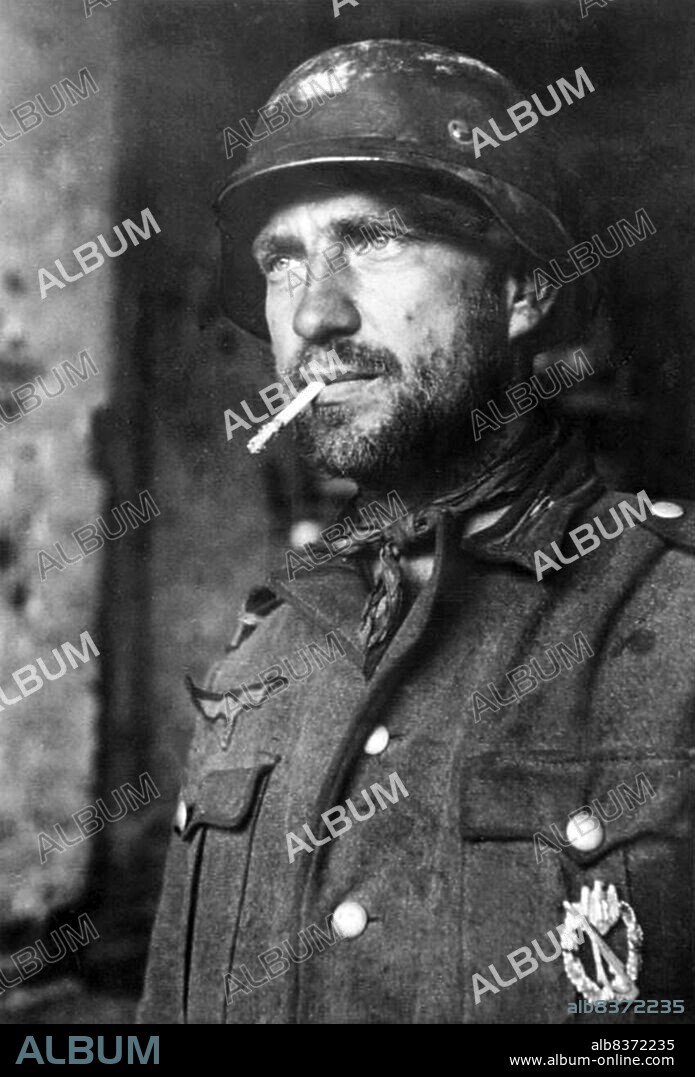The black and white photograph captures a soldier with an air of seasoned weariness. Light-skinned with a serious expression, he has a cigarette hanging from his mouth, its ash unusually long as if he's been lost in thought. His face is framed by a goatee, and he wears a dirty, worn handkerchief around his neck beneath a sturdy military helmet. His fatigues are stained and worn, adorned with patches and an indistinguishable medal on his breast pocket. The background, grainy and out of focus, suggests an old, perhaps professionally taken image. Overlaid across the photo are numerous watermarks reading "album," with additional text in the lower corners: "ALB 837-2235" and "www.album-online.com." This haunting image thus preserves the hard realities of a time long past, immortalizing the soldier’s experienced gaze.